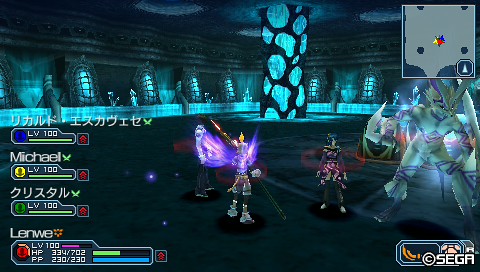The image depicted is a detailed screenshot from a SEGA video game. The bottom right corner prominently displays the "SEGA" logo and a copyright notice. In the top right corner, there is a square mini-map, providing navigation assistance. To its left, white Chinese characters are visible, likely indicating game commands or information. The left side of the screen, starting from the middle and extending downward, showcases various team members' health bars, levels, and names. The bottom-most bar represents the controlling player's character, featuring their hit points, level, and a fully-charged blue meter. The scene is set within a luminescent blue room, adding a mystical ambiance. A character with radiant butterfly wings stands in the forefront, while a transparent figure is seen to the right, adding to the ethereal visual experience.